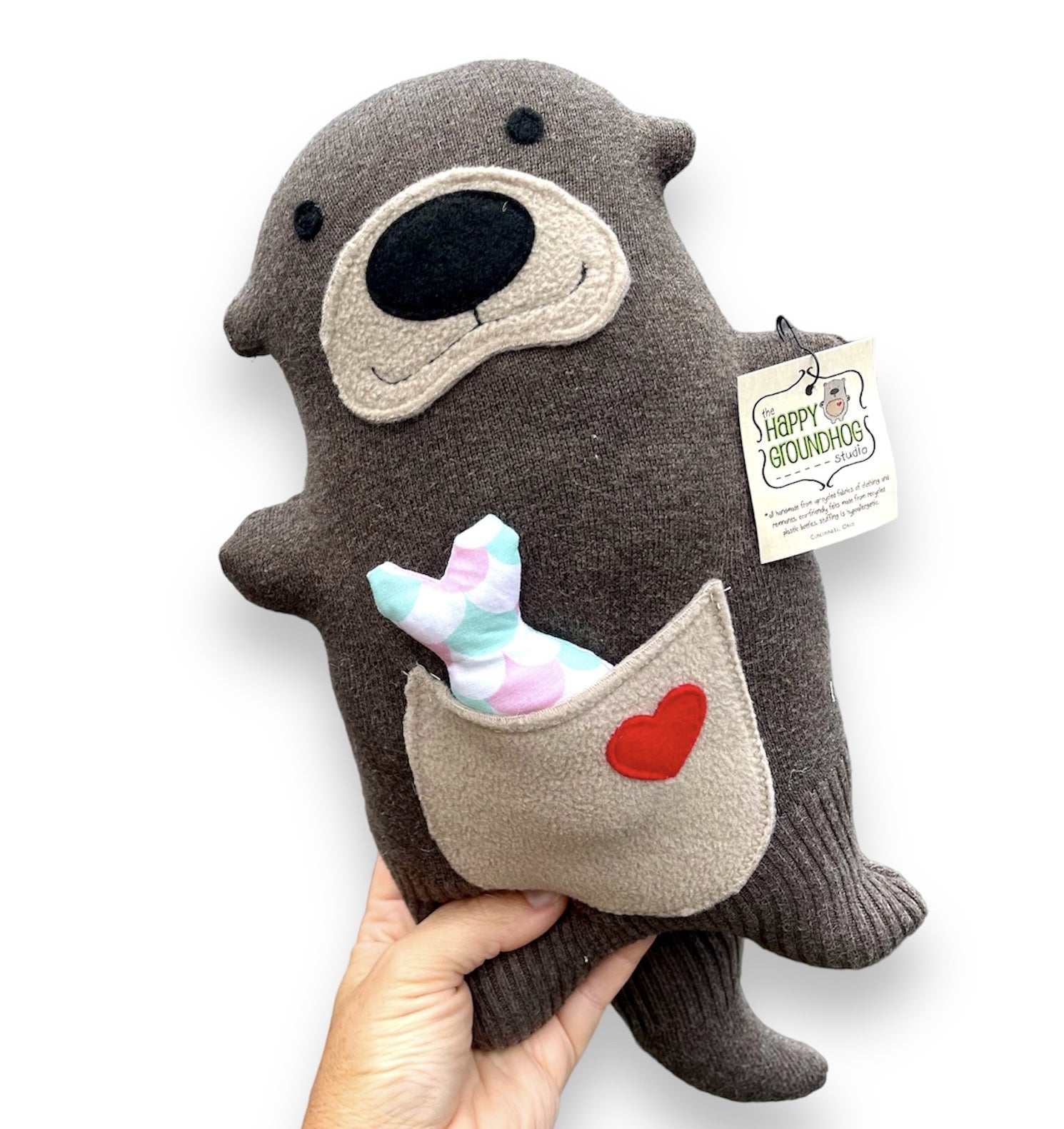This product photograph showcases a commercially-styled plush toy, designed to appeal to young children or babies. Set against a solid white background—common for online shops, listings, or catalogs—the stuffed animal is a cartoonish gray groundhog, made of knit yarn and minky type fur. A human hand, partially visible and presumably off-frame, is holding its bottom left leg. The groundhog features a long gray tail and a tan-colored pouch sewn onto its stomach, adorned with a small red heart in the upper right corner. Peeking out of the pouch is a multicolored fish-shaped stuffed toy in shades of pink, blue, and white, positioned upside down with only its tail showing. The groundhog also has two black felt eyes, a black nose, and a cream-colored area around its nose. A label on its right arm reads "The Happy Groundhog Studio" in green, all capital letters, emphasizing its brand identity. There is also a tag on the arm with the same branding.